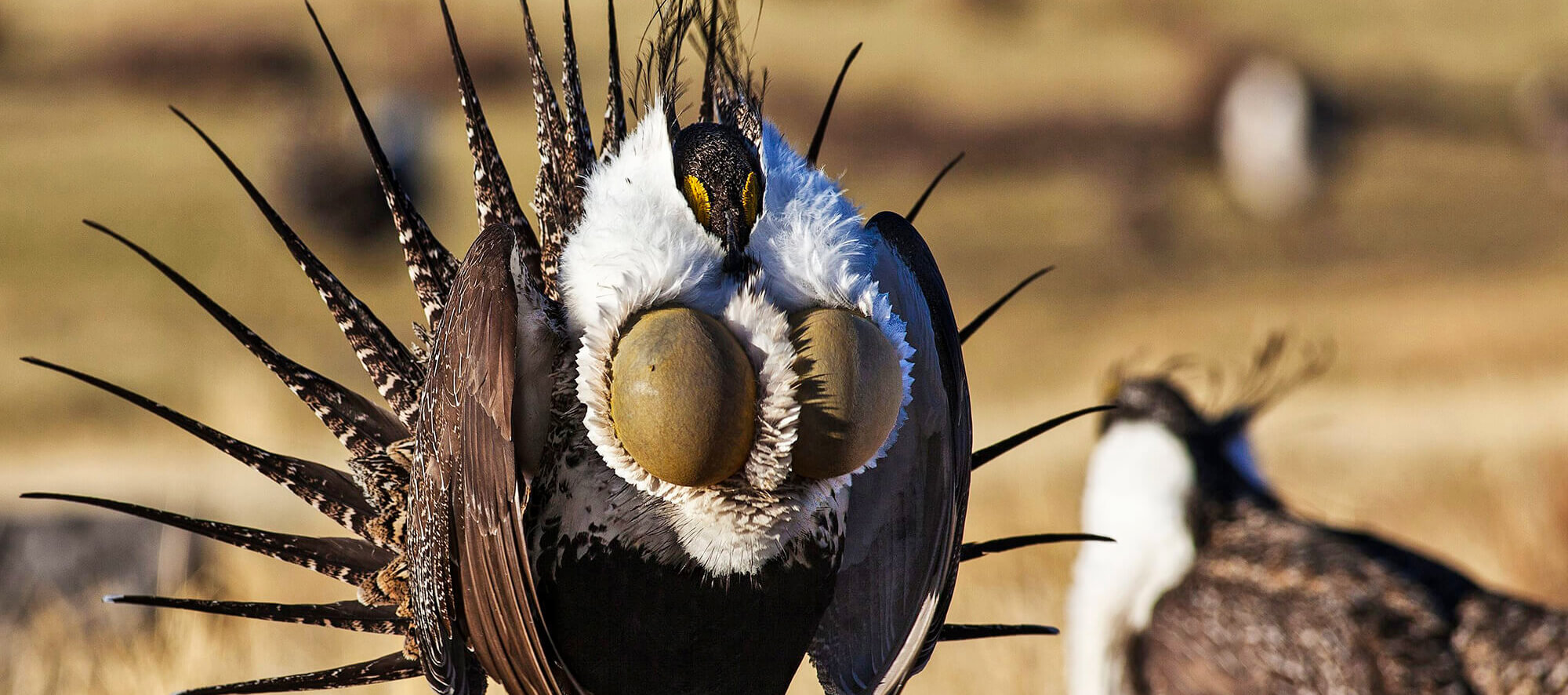This is a detailed photograph of an exotic, large ground bird prominently displayed in the foreground, with another similar bird mirrored in the blurred background. The bird in focus features intricate and vivid feather patterns: its chest is adorned with a striking array of white and black feathers, transitioning into brown wings that curve upwards at the shoulders before cascading down like a long cloak. The tail feathers are notably spiky and fan out in a conspicuous arrangement, showcasing a mix of brown and white stripes.

In the center of its chest, nestled within a plush scarf of white feathers, are two large, coconut-shaped objects that resemble eggs. The bird protectively cradles these "eggs" with its white chest feathers and sweeping wing feathers. Its small, brown head with distinct yellow eye rings peeks out just above this white feathered area, seemingly gazing out with an observant demeanor.

The setting appears to be a prairie, indicated by the fuzzy brown background, giving the impression of a natural habitat. The bird's posture and feather arrangement suggest a sense of vigilance and care, emphasizing its exotic and somewhat mysterious allure.